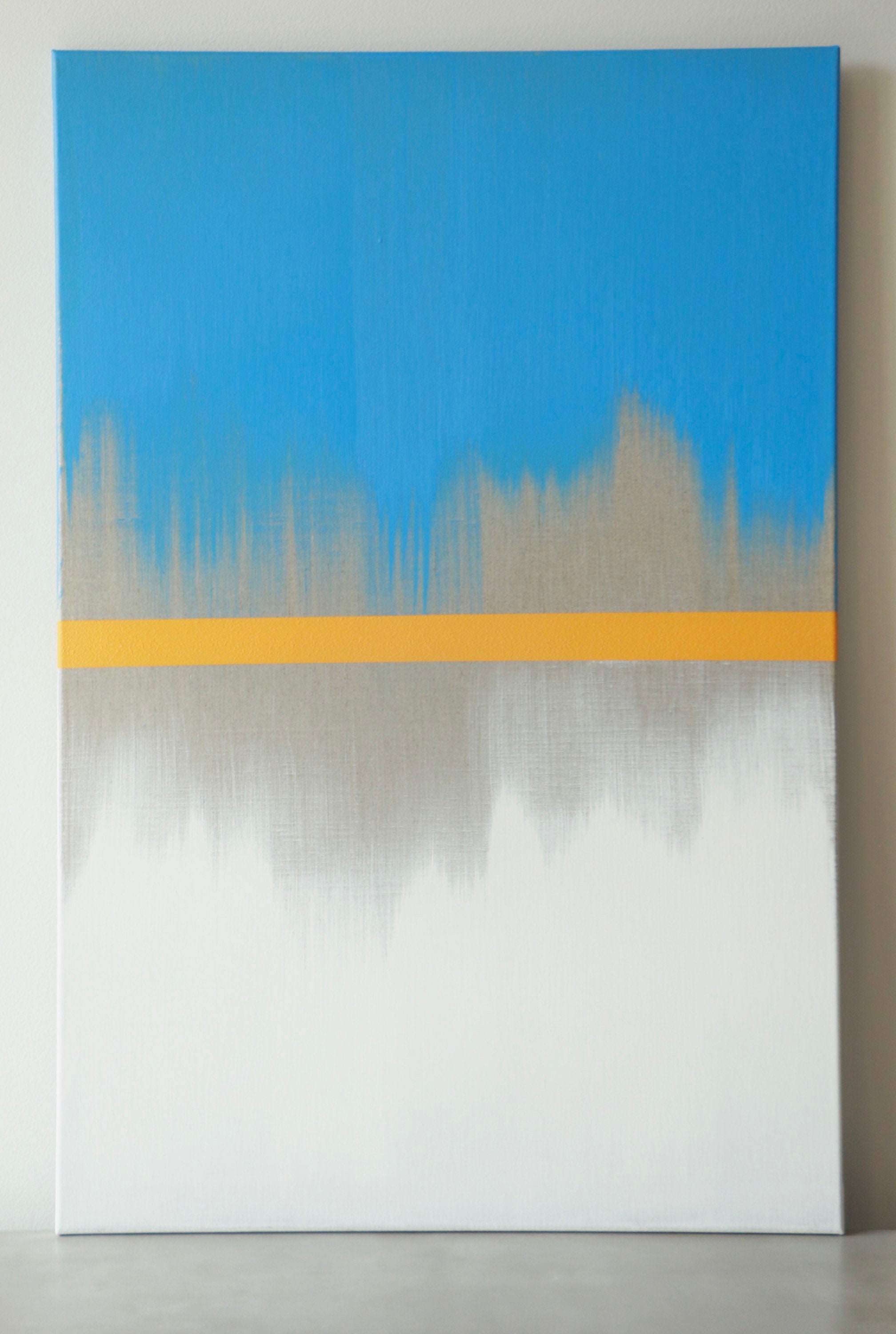The image showcases a vertically rectangular, abstract canvas art piece, leaning against a white wall on a white floor. The canvas features a range of colors and textures: the top third is predominantly a turquoise blue, subtly blending into light brown and grayish-white brushstrokes. A solid yellow vertical line runs through the middle, dividing the composition. Below this line, the artwork transitions into more white splashes and culminates in a chalk-white bottom section. The painting is not framed but wrapped over a frame, emphasized by the shadow on the right, and there's a reflective quality to the glossy floor beneath it.